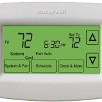In this close-up image of a thermostat, only a portion of the device is visible, suggesting the photo was taken at a close range and possibly cropped. The thermostat, predominantly crafted from white plastic, prominently displays the brand name "Honeywell" at the top. The central feature of the device is a green and black LCD screen that emits a gentle glow, likely due to backlighting. The screen appears to have touch controls, with clearly visible up and down arrows on the right side for adjusting temperature settings. Additional buttons and arrows are located at the bottom of the screen, but their labels are too out-of-focus to be discernible. The thermostat display reads "72," probably indicating the current room temperature, and shows a time of "6:30," though the designation of AM or PM remains unclear due to the blurriness of the image.